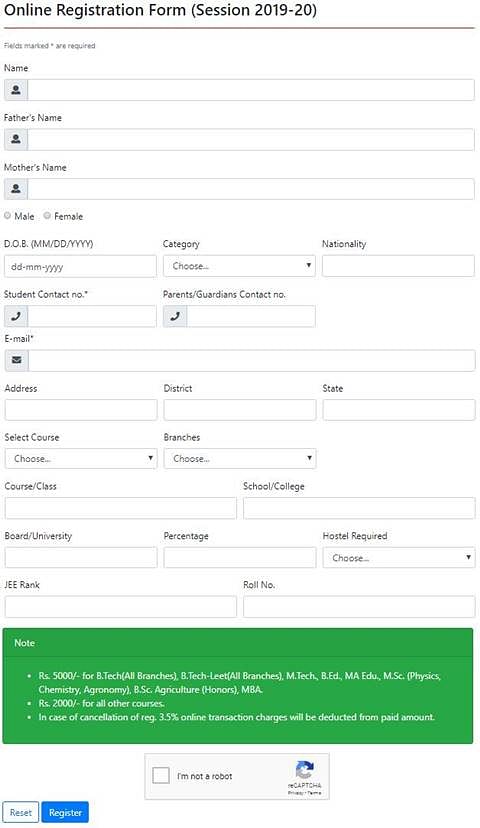In the image set against a pristine white background, we observe a detailed screenshot of an online registration form for the academic session of 2019-2020, positioned in the upper left corner. At the top, it mentions that fields marked are required in small gray text. The form's first field, labeled "Name," is prominently displayed with a text box for input below it. Following, we find boxes for "Father's Name" and "Mother's Name," each with respective labels.

Below these fields, there are two radio button options labeled "Male" and "Female" for selecting the gender of the registrant. The subsequent line is marked for inputting the "Date of Birth," formatted as month, date, and year, and includes a corresponding text box. To the right of the date of birth field is a category section with a pull-down menu, followed by a space for indicating nationality.

Beneath these fields lies a section for the "Student's Contact Number," which is denoted with an icon of a phone. Adjacent to it on the right is space for the “Parent/Guardian's Contact Number,” also accompanied by a phone icon. This is followed by a field for "Email Address."

Moving further down, the form has fields for "District" and "State," and provides pull-down menus to "Select Course" and "Branches," allowing for specific selections. The layout is organized and systematically arranged for easy use and readability.